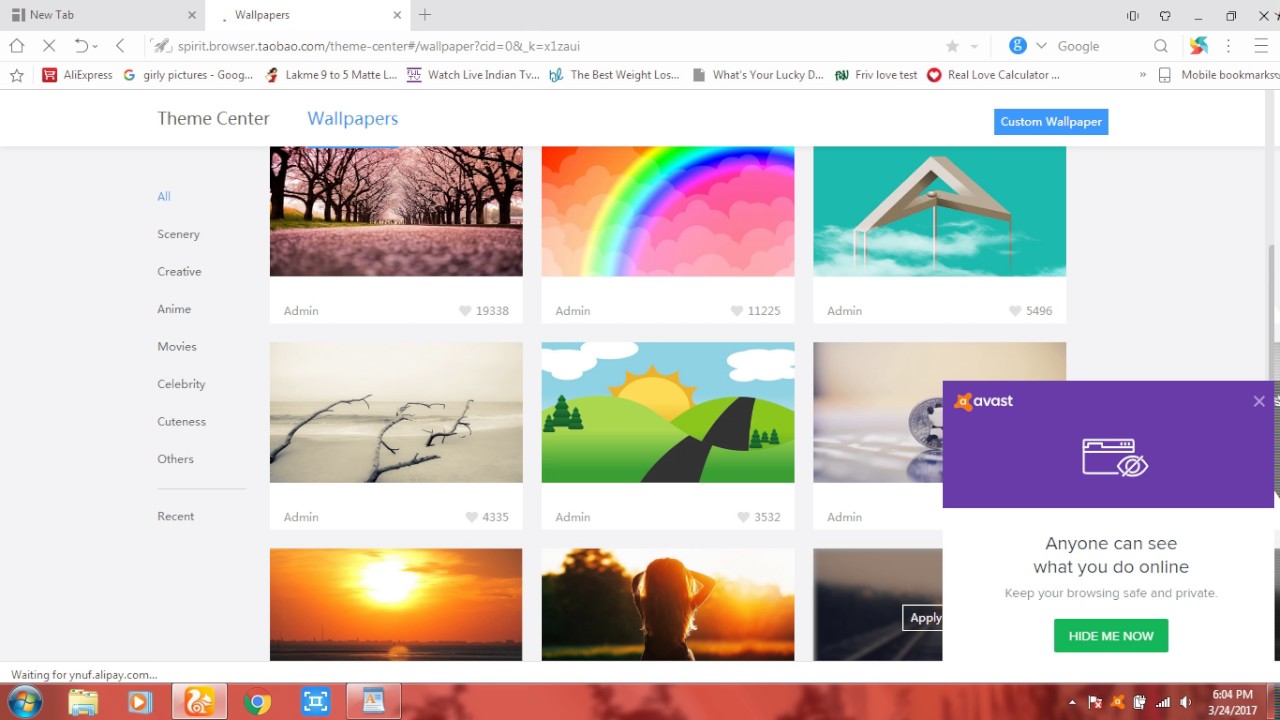A computer screen displays the Microsoft Edge browser, open on a Windows 7 operating system. The browser has two tabs open: one labeled "New Tab" and the other "Wallpapers," leading to a webpage on taobao.com within the theme center section dedicated to wallpapers. The site showcases a variety of attractive wallpapers, including a picturesque dirt path leading up to a house, framed by trees with vibrant purple or pink blossoms. Other images feature a combination of natural and digital artistry, such as a sky adorned with a rainbow and pink clouds, a geometric triangle suspended in the sky, a serene beachscape, and a sunlit cartoon-like meadow. Additionally, a stunning sunset, and an image of a girl gazing into the sunset are also visible. In the bottom-right corner of the screen, a notification from a vast antivirus software has appeared, likely prompting the user to purchase the software.